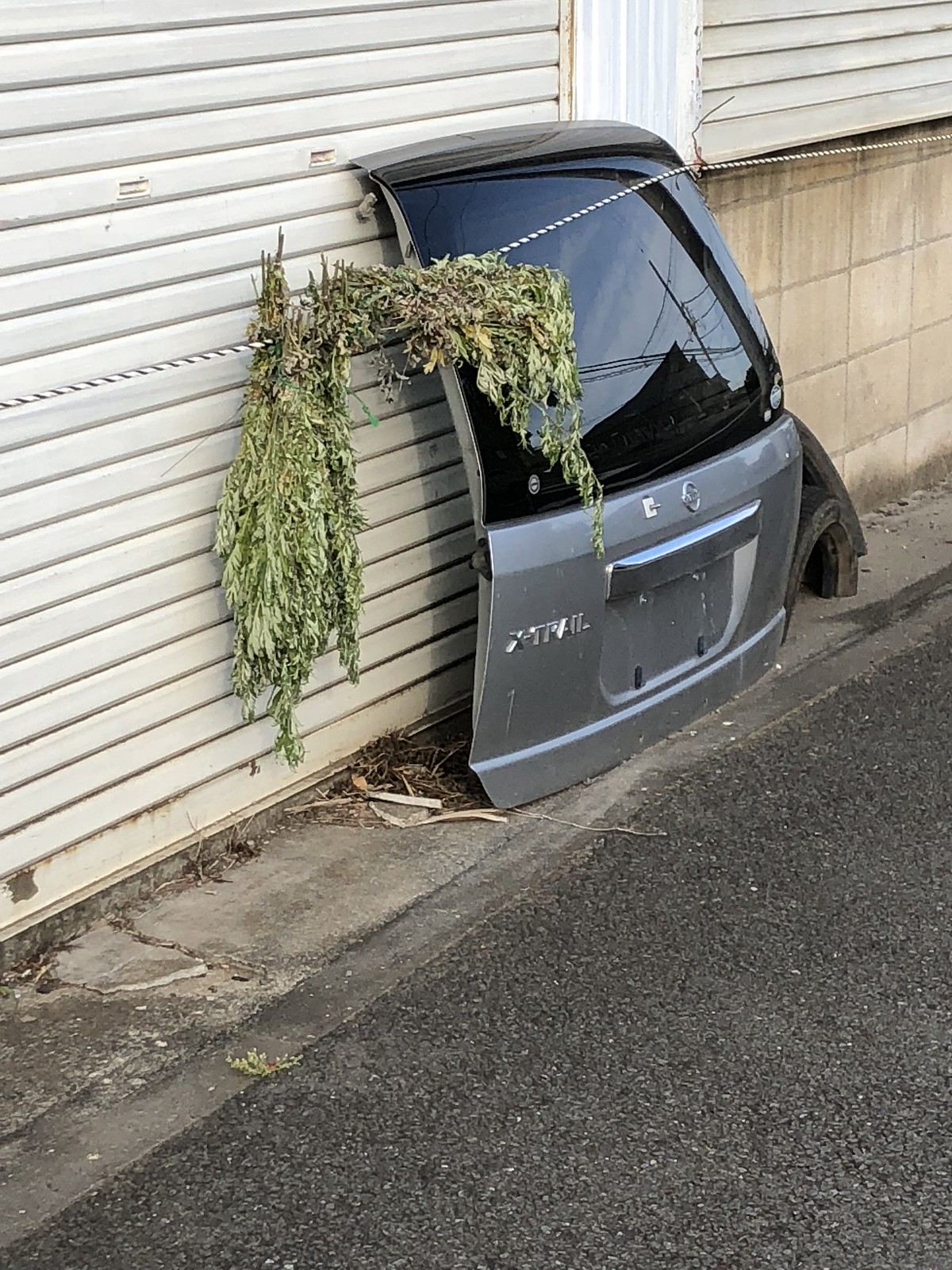In this daytime outdoor photograph, a detached gray car door, possibly from a hatchback or van, is leaning against a building facade that features both concrete and brick elements. The door, which lacks its license plate, displays the faint text "trail" and the partial marking "4X." A white rope secures the door to the building, with green bush branches entwined in the rope. Set on a narrow sidewalk against a dark gray street, the door is juxtaposed between two wall sections: one lighter concrete with little beams and the other darker gray. The scene is devoid of people but rich in urban and natural contrasts.